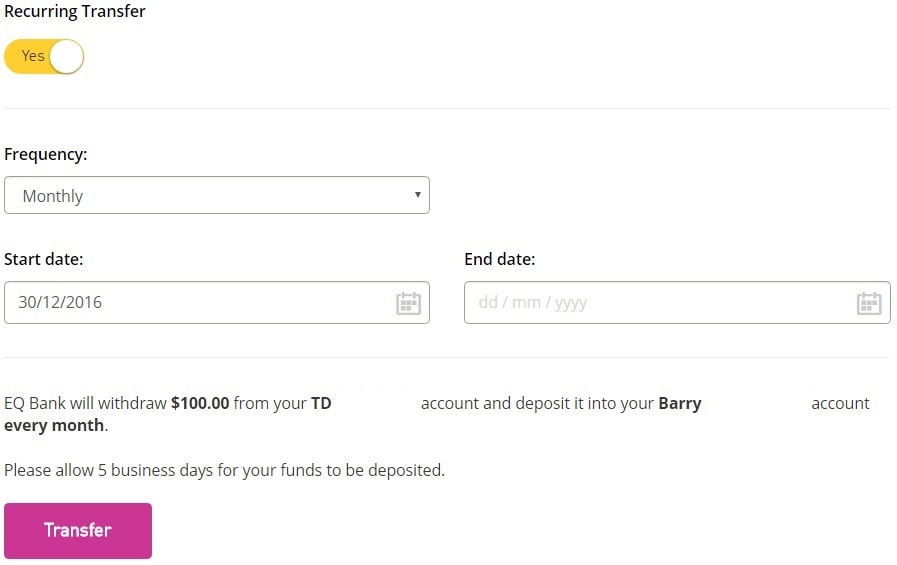Set against a clean white background, this image showcases several key elements of an online transfer form. In the upper left corner, there is a bright yellow toggle button labeled "Yes." Directly above it, black text reads "Recurring Transfer." Beneath the toggle button, there is the word "Frequency" followed by a dropdown menu set to "Monthly." 

The next section down features the label "Start Date" with an adjacent text box filled with the date "30-12-2016." Below this text box, an important notification in black text states: "EQ Bank will withdraw $100 from your TD every month. Please allow 5 business days for your funds to be deposited."

At the bottom of the image, there is a prominent purple action button labeled "Transfer." On the right side of the screen, there is an "End Date" section with an empty text box accompanied by a small gray calendar icon. Below this section, additional text specifies that the funds will be deposited into your Barry account.

This detailed layout clearly outlines the process and settings for scheduling a recurring financial transfer, emphasizing key functionalities and instructions.